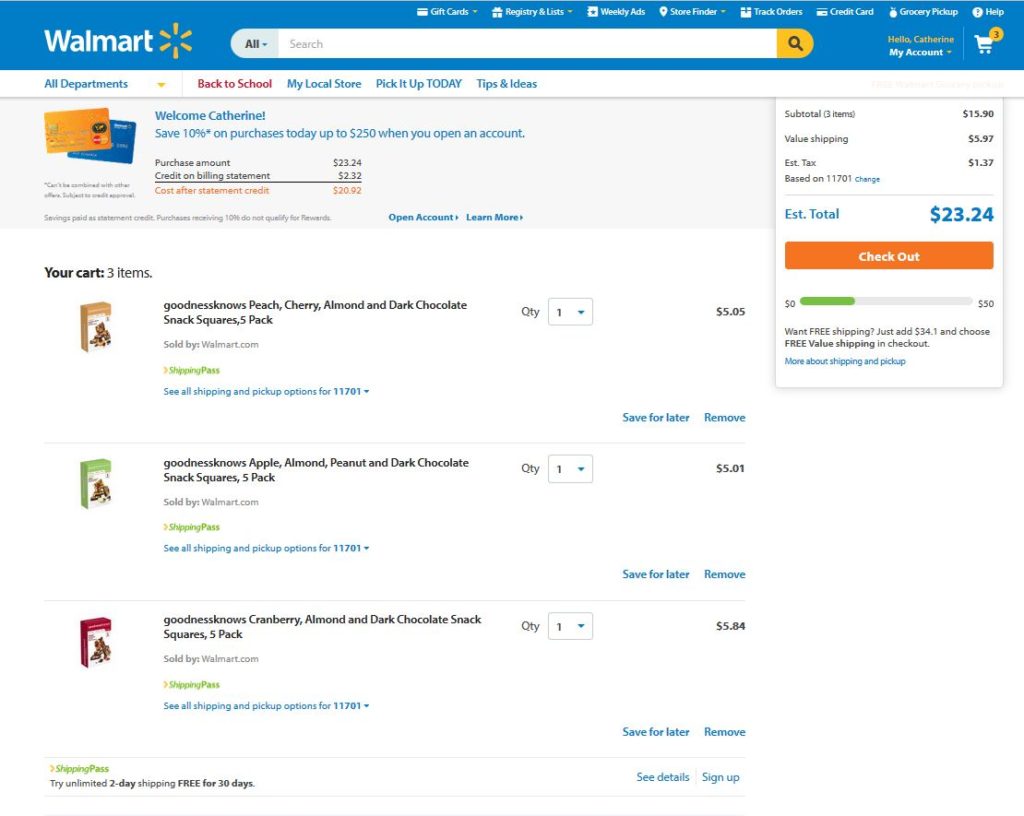The image is a screenshot from the Walmart.com website, featuring a design that appears to be from a few years ago, characterized by older graphics and layout. At the top of the page, the Walmart logo is prominently displayed, with a centered search bar and user interface options such as 'My Account' and a shopping cart icon on the right.

Above these primary elements, there is a navigation bar with various small-text menu options. Below this, a white bar runs across the width of the screen, housing a 'Departments' button alongside different shopping categories. Within the main section of the webpage, the user's shopping cart is shown, containing three items, each a different flavor of snack or candy. The items, which resemble trail mix bars, have images to their left.

In the upper right corner of the main section, just below the Walmart heading, the shopping cart details are displayed. The total cost of the items in the cart is $23.24. Additionally, there is a checkout button, allowing the user to proceed with their purchase.